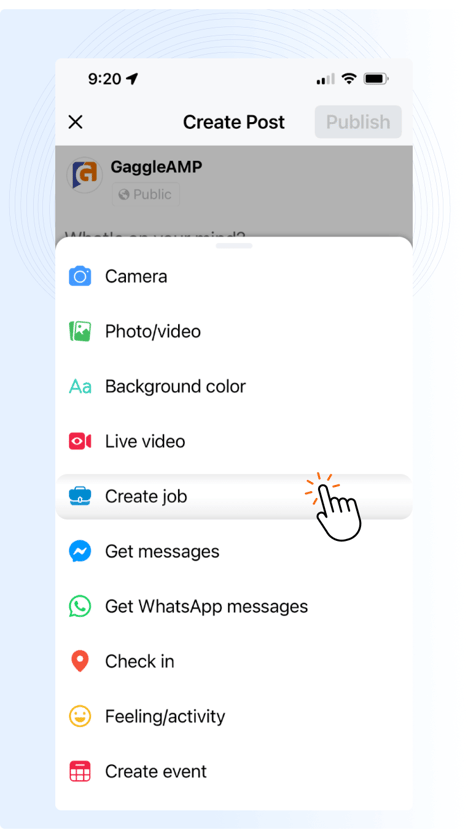The image features a light blue background with a white drop at the top, displaying the number '920' and an arrow pointing to the upper right. Adjacent to this, there are battery icons and other standard interface elements. In the upper portion, there's an 'X' button and a 'Create Post' label, followed by a small gray button labeled 'Publish.'

Prominently, there is a dark gray section containing a blue and orange icon with the letter 'G' and the text "Gaggle Amp," marked as 'Public.' Below this, there is partially obscured text indicating more content.

On a white background, a series of icons are arranged: 'Camera,' 'Photo/Video,' 'Background Color,' 'Live Video,' 'Create Job' (which is highlighted), with a hand icon indicating interaction, 'Get Messages,' 'Get WhatsApp Messages,' 'Check In,' 'Feeling/Activity,' and 'Create Event,' each accompanied by its respective icon.